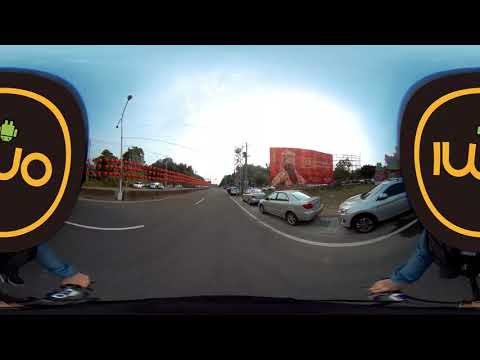The image captures a mirrored, panoramic view of a street under bright daylight. The focal point is a person riding a bicycle down a two-lane, gray asphalt road marked with white lines, both solid and dotted. This individual wears a blue long-sleeved garment and appears partially obscured by a censoring icon—a black circle with a yellow interior featuring the letters "IWO" and a small upside-down green Android figure. On the peripheral edges of the image, you can see the person's hands gripping the bicycle's handlebars.

Several gray or silver sedans and SUVs are parked along the right side of the road. A towering red billboard with indistinguishable advertisements and possibly a figure, perhaps a celebrity or political persona, looms in the background. The sky above is a bright blue with traces of overcast clouds, adding to the luminosity of the scene.

Additional elements include street lanterns and electrical wires, along with some red balls suspended on wires forming a fence on the left side. In one corner, a person on a bicycle or moped can be noticed, further enhancing the dynamic feel of the image.